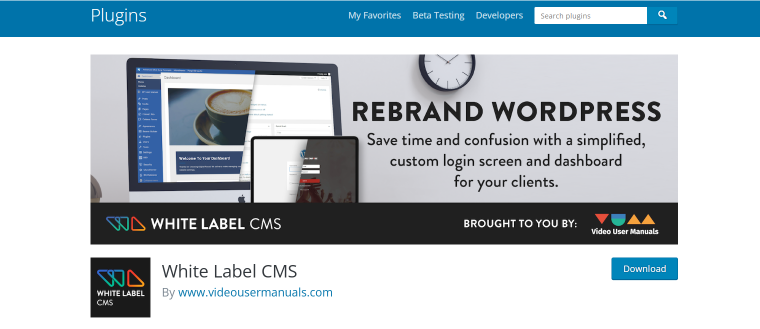Here is a cleaned-up and detailed descriptive caption for the image:

---

The image is a screenshot from a webpage featuring a distinctive blue bar at the top. In the upper left corner of this bar, "Plugins" is displayed in white text with a capital 'P'. To the right of this, there are headers reading "My Favorite Beta Testing Developers," also in white text. In the upper right corner, there is a white search box labeled "Search Plugins," accompanied by a blue button featuring a white magnifying glass.

Below this top bar, the main body of the webpage is visible. On the left side, there is an image of a computer screen displaying a picture of a coffee mug and a blue menu on the left side. Adjacent to the screen on the right is an analog clock with a black outline, a white face, and black hands.

Centered at the top of the main content area, bold black text reads "REBRAND WORDPRESS." Below this heading is a subheading stating, "Save time and confusion with a simplified custom login screen and dashboard for your clients."

Beneath this section, there is a black bar containing the text "White Label CMS" alongside a logo composed of two blue triangles pointing to the upper right and one red triangle pointing to the lower left. The text also mentions that the service is "Brought to you by Video User Manuals," accompanied by additional design elements, including a red triangle, a green and blue semicircle, and two orange triangles.

In the lower left corner, "White Label CMS" is displayed in white text within a black box featuring three triangles. To the right, it reads, "White Label CMS by www.videousermanuals.com." In the lower right-hand corner, there is a blue "Download" button.

---

This descriptive caption provides a clear and comprehensive overview of the webpage layout and content within the screenshot.